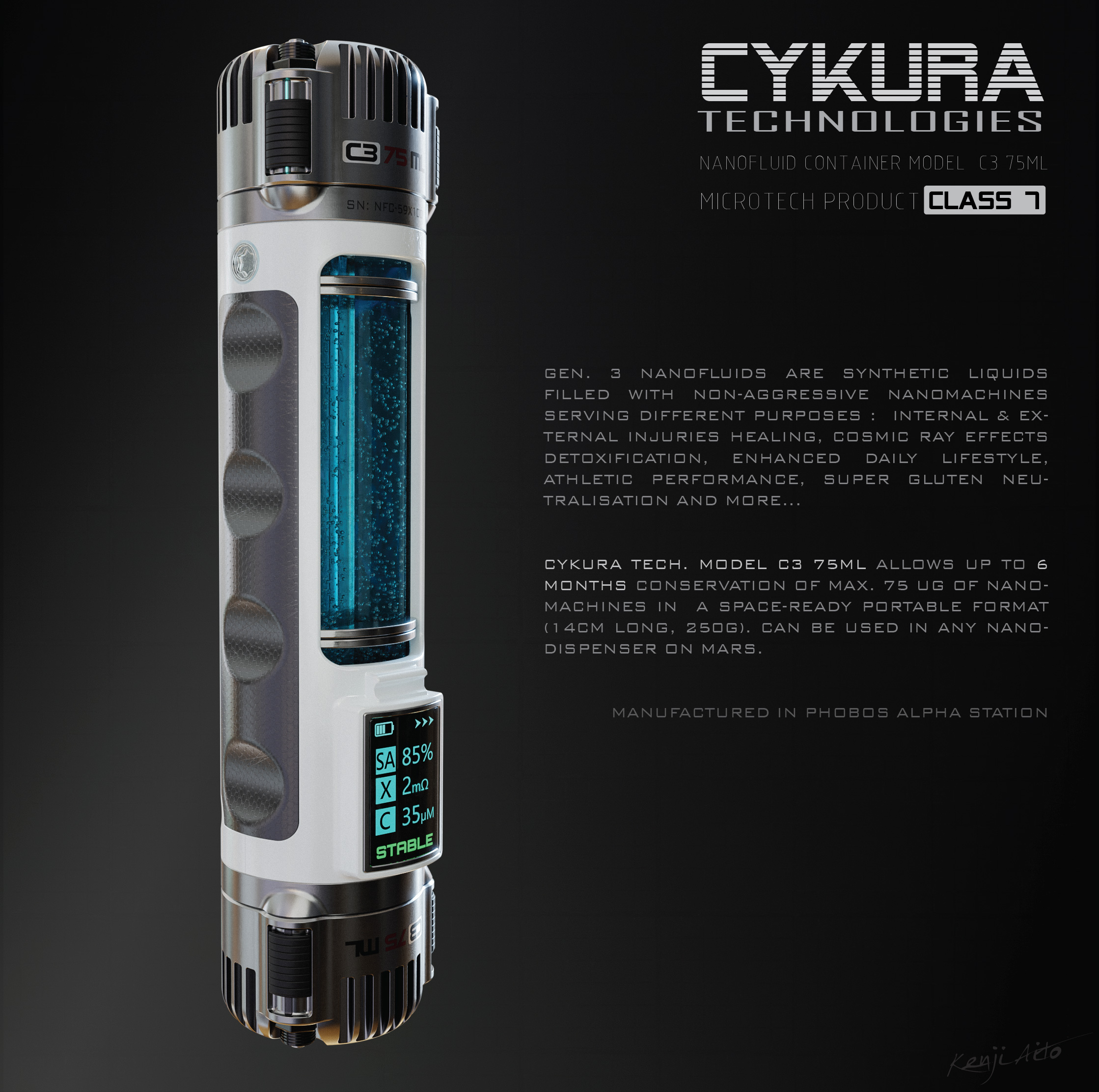This is an advertisement featuring a futuristic, science fiction device from Sykura (C-Y-K-U-R-A) Technologies. The background is predominantly black with a subtle white-gray gradient emerging from the bottom left corner. Dominating the left side of the image is a slender, cylindrical object resembling a baton or flashlight. The device has a sleek white body with silver caps at either end, which incorporate vent features, and an eye-catching blue liquid visible through a central window. The device is equipped with an electronic display near the bottom, showcasing details such as "SA 85% X 2 milliliters" and "C," along with a battery charge indicator.

In the upper right corner, the company's name, Sykura Technologies, is prominently displayed in large white text. Below it, additional information describes Generation 3 Nanofluids, synthetic liquids infused with nanomachines designed for various health applications, including healing internal and external injuries, counteracting cosmic ray effects, detoxification, and enhancing daily lifestyle and athletic performance. The text further mentions that this advanced Class 7 Microtech Product, Model C375ML, is manufactured in Phobos Alpha Station.